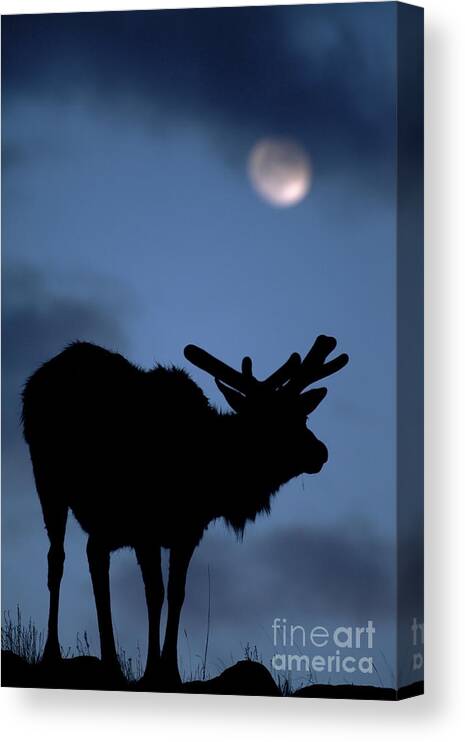The image is a detailed nighttime scene, likely depicted on a canvas wall art or possible book cover, with predominant shades of blue and darker blue. It features a striking black silhouette of a large, four-legged animal with shaggy fur, two ears, and prominently antlers, identified either as a moose or an elk. The animal stands in profile atop a hill or rocky patch surrounded by indications of grass and weeds. The sky behind the animal is adorned with wispy, dark blue to gray clouds, partially obscure a glowing white moon. The landscape's silhouette, along with the animal's detailed form, contrasts sharply against the illuminated night sky. A light-colored watermark reading "Fine Art America" is visible in the bottom right-hand corner of the image.